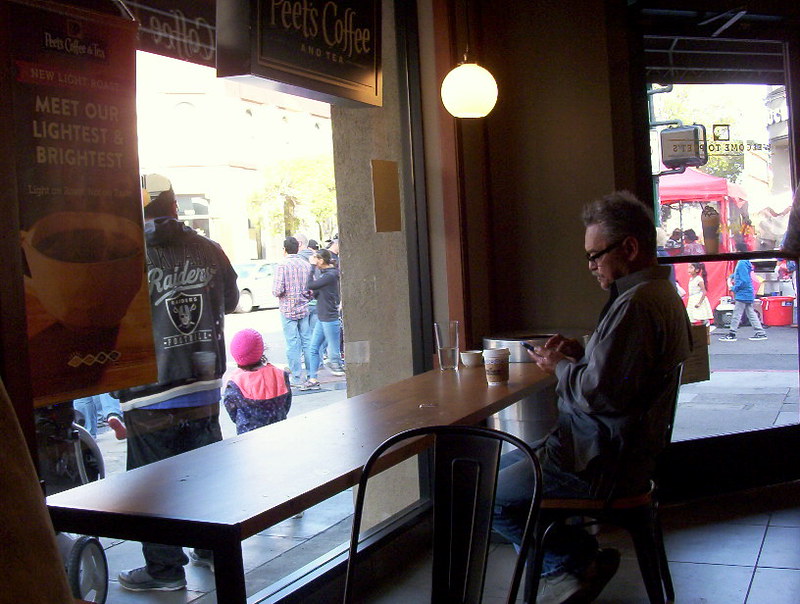The photograph captures the interior of a cozy coffee shop. At a wooden table near the center of the image, a middle-aged man dressed in a gray jacket, jeans, and gray shoes is seated, engrossed in his phone while sipping coffee. He also wears glasses. The table holds a coffee cup and a glass filled with water, along with some other miscellaneous items. The walls of the coffee shop are adorned with informational banners about coffee, and a notable sign in the upper left corner reads, "Peace, Coffee, and Tea."

To the left, there is a large glass window offering a view of the bustling street outside. Through this window, you can observe a man in a gray Oakland Raiders jacket standing next to a little girl. They are part of the vibrant street scene, where various people are either standing or walking around, and vehicles are also visible. On another wall, a glass door provides another glimpse of the outside world, enhancing the coffee shop's inviting and interconnected atmosphere.